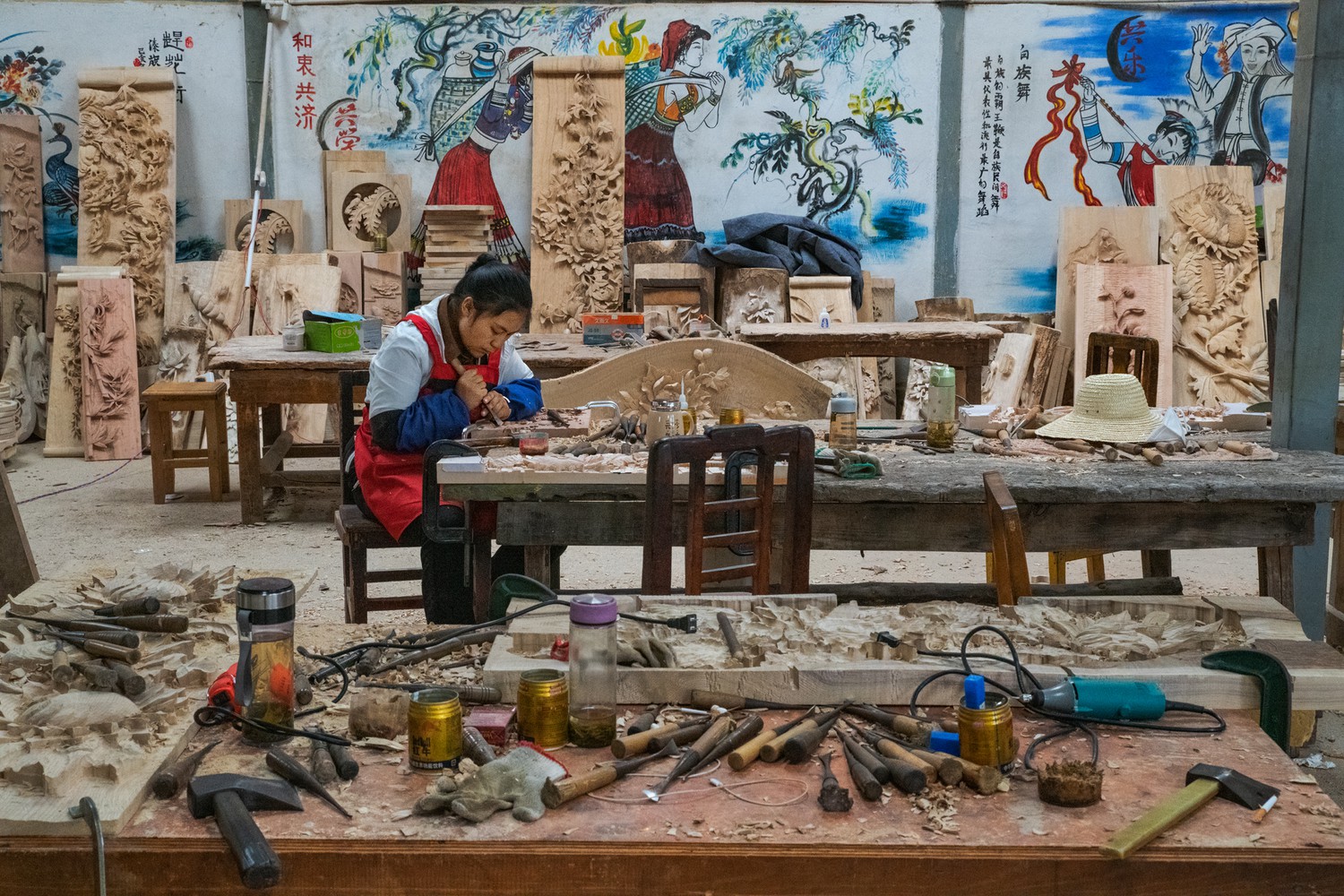In this realistic photograph, an Asian woman is meticulously engaged in woodworking, using a hand chisel to carve a piece of wood on a cluttered wooden table. She is dressed in a red apron over a blue shirt, with a long-sleeved dark blue shirt underneath, and her dark hair is pulled back into a ponytail. The foreground is filled with various tools like chisels and hatchets, water bottles, remnants, and unfinished wooden blocks. Surrounding her workspace are additional woodworking materials and partially completed projects. The background is adorned with intricate wooden reliefs and watercolor paintings depicting Asian imagery, such as bonsai trees, a tiger, Chinese warriors, flowers, and scenes of people walking with baskets. Japanese handwriting and traditional paintings embellish the walls, enhancing the cultural atmosphere of the workshop.